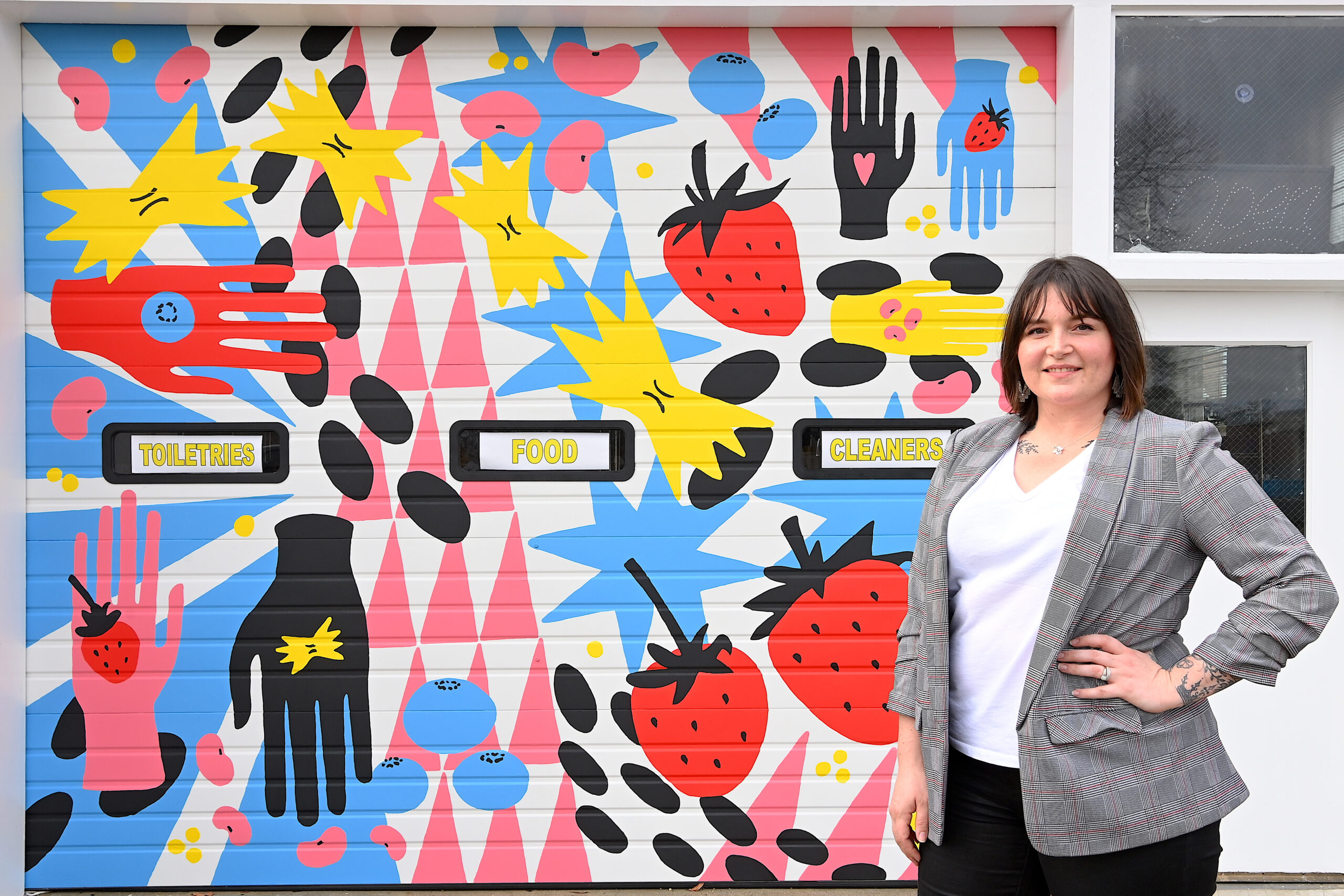A woman stands confidently before a vibrant, colorful mural painted on a surface resembling slats, possibly of a garage door. She wears a semi-casual gray business suit over a white V-neck undershirt, accessorized with a necklace and visible tattoos on her chest and hand. Her short hair grazes her shoulders and she has a pleasant smile directed at the camera, with one hand resting on her hip.

Dominating the composition behind her, the mural bursts with a lively array of colors—red, light pink, yellow, light blue, and black, set against a primarily white background. Three prominent words, "toiletries," "food," and "cleaners," are inscribed within black squares and white-bordered sections at the center of the artwork.

The mural features a plethora of detailed, interwoven shapes and motifs. Blue and pink triangles create dynamic patterns on the left, while light blue, distorted star shapes seem to explode in a vibrant swirl. Scattered throughout are illustrations of strawberries, blueberries, and what appears to be yellow pasta. Black ovals add to the energetic flow, swooshing toward the bottom right.

A notable element is the assortment of hands in different colors—pink, blue, and black—each holding distinct objects such as a red strawberry, a pink heart, and a yellow ribbon or pasta. These hands, some also embellished with shapes in their centers, add a sense of interaction and community to the mural's theme. The backdrop of the mural's spirited design subtly complements the woman’s poised presence.